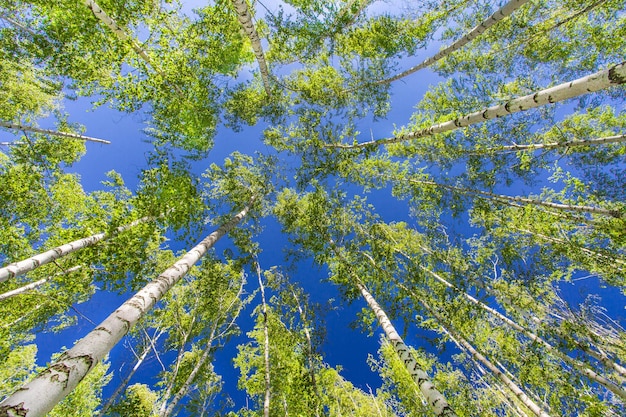This image captures an immersive view from the forest floor, where one finds themselves at the base of incredibly tall, white-barked birch trees. The perspective is as if lying on the ground, looking straight up into the sky. The trees encircle the viewer, with their thin yet towering trunks spaced just enough to allow glimpses of the vibrant blue sky, unmarred by clouds. The green leaves at the tops of the trees, more concentrated towards the upper branches, suggest that the season is spring or summer. The sky shifts from a saturated medium-to-dark blue at the base to a lighter, almost hazy whitish blue towards the top, creating a striking and somewhat surreal contrast against the stark white and black-striped bark of the birches. The overall scene conveys the tranquility of nature with an emphasis on the towering presence of the trees and the pristine clarity of the sky, beautifully captured with high detail.